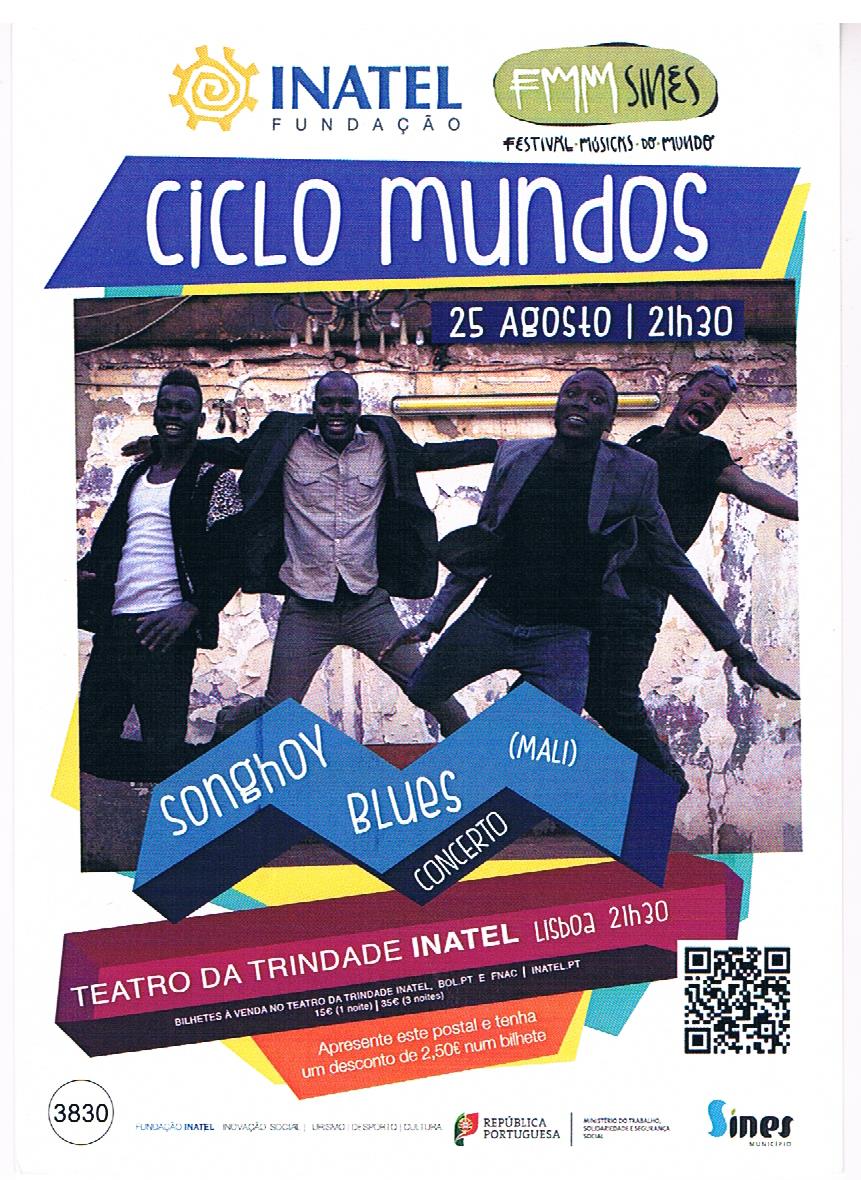This vibrant advertisement poster for the Ciclo Mundos festival showcases an energetic photograph of four black men, aged 25 to 30, mid-jump and smiling warmly. These men, identified as the musical group Songhoi Blues, each exhibit their unique style. The man on the far left sports a white tank top paired with a black blazer and black jeans. Beside him, another member wears a brown or pink button-up shirt under a blazer, complemented by grey jeans. The third man dons a black tank top with a blue blazer and blue jeans, while the person on the far right is casually dressed in a black t-shirt and blue jeans. 

Above the image, logos associated with the event are visible, including one resembling a sun, labeled “Inetel Fundacao.” The text details, mostly in Spanish, state "Ciclo Mundos 25 de Agosto, 21H30," indicating the event starts at 9:30 PM on August 25th. Additional logos, including one representing the Republica Portuguesa, are also present. There is a QR code intended for more information, and the poster advertises their concert venue at TITRO.TRINIDAD INATEL LISBO. The image is set against a backdrop of a cement wall, underscoring the casual yet exciting atmosphere of the festival. The numbers 3830 appear within a circle at the bottom left of the image, adding another layer of detail to the promotional material.